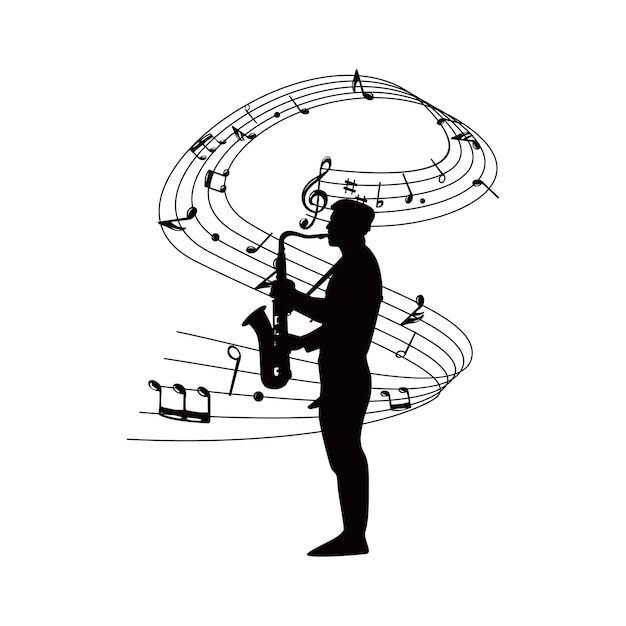A black and white illustration depicts a silhouette of a man playing a saxophone. Positioned in profile, he faces the left side of the image, his form entirely rendered in black, leaving no visible details of his face, clothes, or shoes. Behind him, a musical staff winds and swirls in a dynamic S shape, adorned with various musical notes that appear to dance and spiral around him, adding to the sense of movement and rhythm in the scene. The overall composition captures the essence of music in motion, with the figure immersed in the act of playing his instrument.